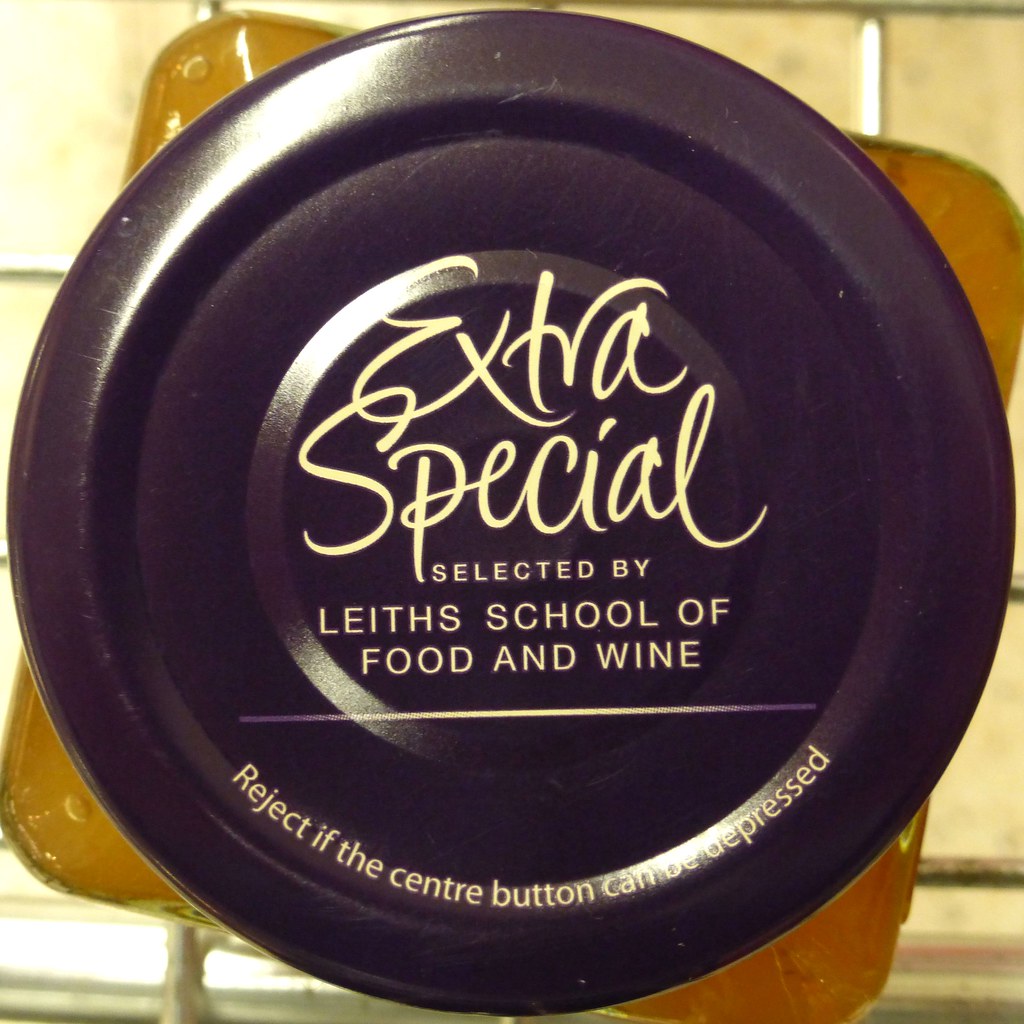The image depicts a top-down view of a circular black lid belonging to a bottle or jar, possibly containing a beverage or culinary ingredient given the association with Leith's School of Food and Wine. The lid features large, elegant cursive text that reads "Extra Special" in gold or yellow lettering. Beneath this, in smaller, sans-serif all-caps text of the same color, it states, "Selected by Leith's School of Food and Wine." At the bottom of the lid, a warning in capital letters advises, "REJECT IF THE CENTER BUTTON CAN BE DEPRESSED," with "center" spelled in the British style ("centre"). The contents of the bottle appear to be a golden, honey-like liquid. The background of the image hints at a light yellowish surface, possibly a table, on which the bottle is placed.